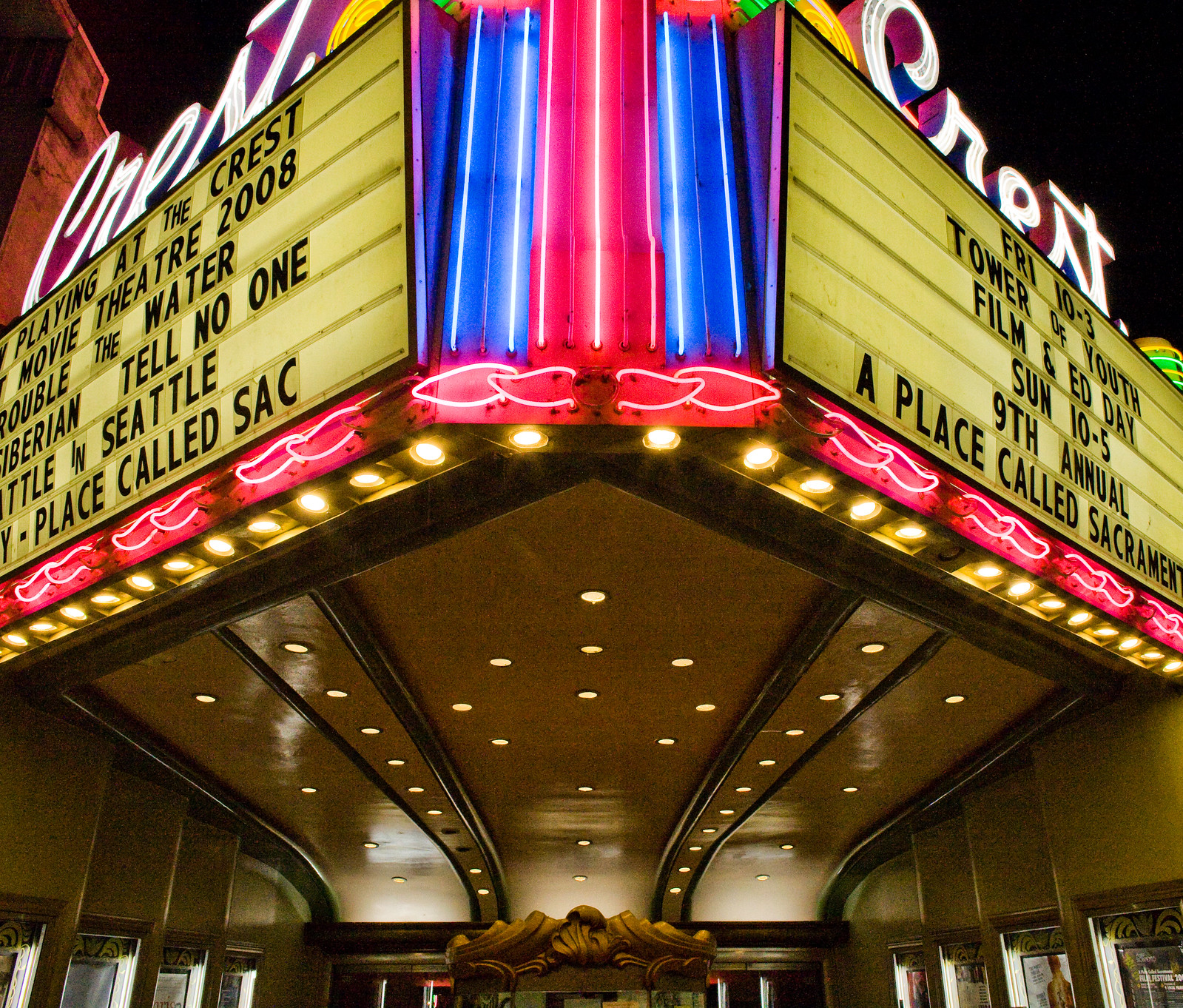This image showcases a close-up of the exterior of a movie theater, reminiscent of a venue for a Broadway musical, adorned with vibrant red and blue lights. The brightly illuminated marquee displays white cursive lettering at the top and beige-colored signs with black text on both sides. The text on these signs reads: "Playing at the Crest Movie Theater 2008, Something in the Water, Tell No One, Something in Seattle, Place Called SAC." The right-hand side sign further details event timings: "Friday 10 to 3, Tower of Youth, Film and Ed Day," and "Sunday 10 to 5, 9th Annual, A Place Called Sacramento." The image, filled with an array of colorful lights, suggests a bustling atmosphere outside the theater. Some text appears slightly cut off, indicating the photograph captures the marquee from a dynamic angle, emphasizing the detailed list of upcoming showings and events.